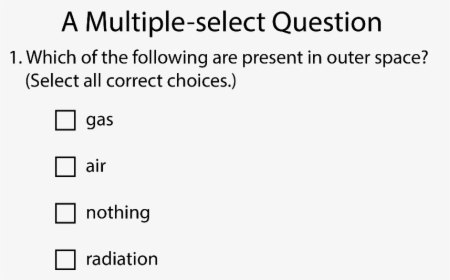In this black-and-white image, we see an educational page designed to test knowledge about outer space. At the top of the page, there is a bold, prominent heading that reads: "Multiple Select Question." Below this heading, there is a label indicating "Number One," followed by the question: "Which of the following are present in outer space? Select all correct choices." 

Under the question, there are checkboxes aligned vertically next to four options: 
1. Gas
2. Air
3. Nothing
4. Radiation

The format is repeated to emphasize the instructional nature of the question: "Multiple Select Question. Number One. Which of the following are present in outer space? Select all correct choices. Gas, Air, Nothing, Radiation." The layout is simple yet clear, with each option easily distinguishable for selection.